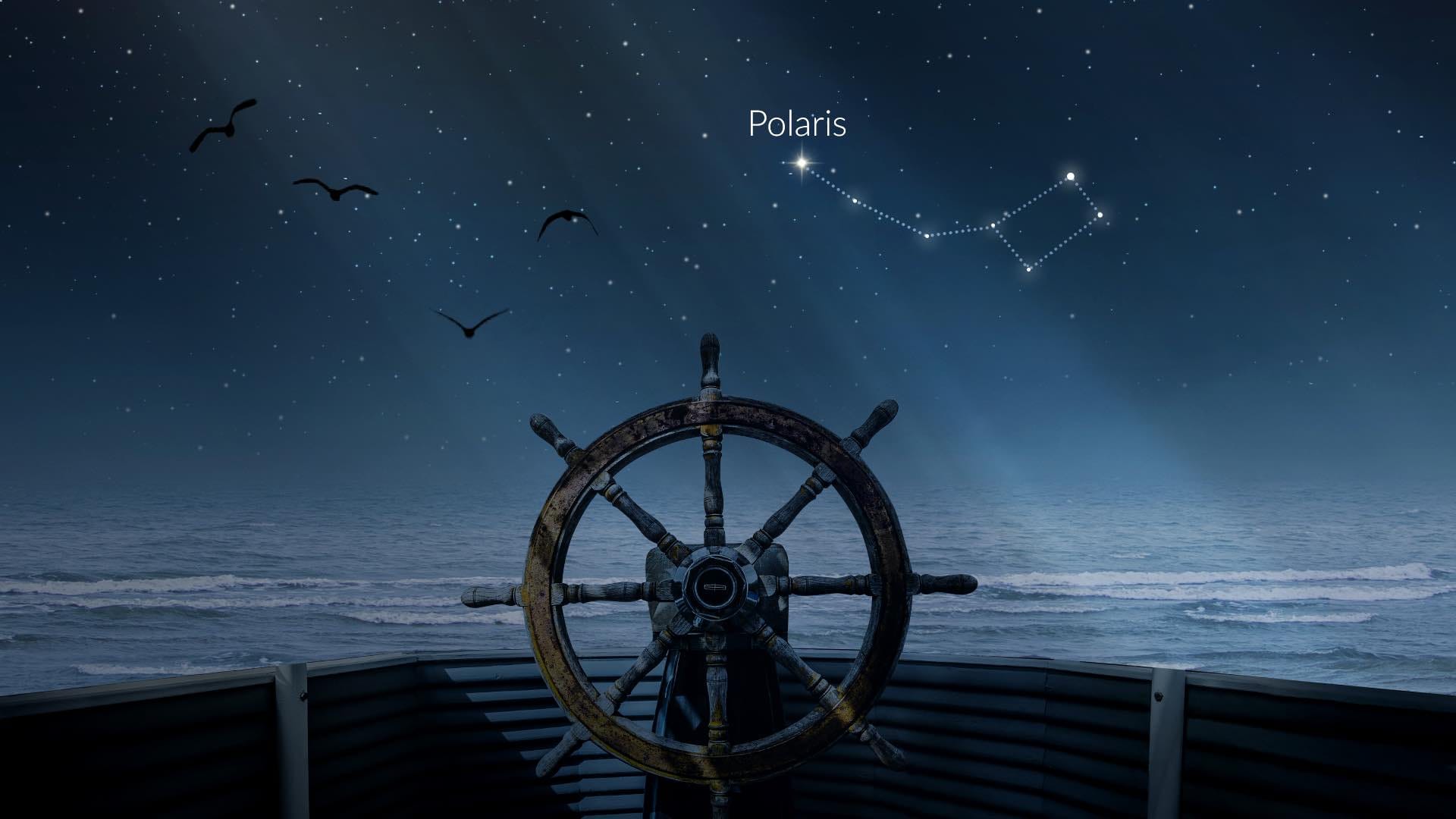The image depicts an artful nighttime scene from the perspective of the bow of a ship, showcasing an old-fashioned steering wheel with handles extending outward. The ship is surrounded by the vast ocean, where white-capped waves ripple below. The sky transitions from a light gray-blue hue near the horizon to a deeper twilight blue as it ascends, filled with numerous stars of varying shapes and sizes. Four silhouetted birds can be seen loftily flying in the top left corner. Prominently featured is the constellation Polaris, with white lines connecting the stars to form a ladle-like shape or dipper. The bright star at the center has "Polaris" written in white above it, highlighting its significance in the celestial display.